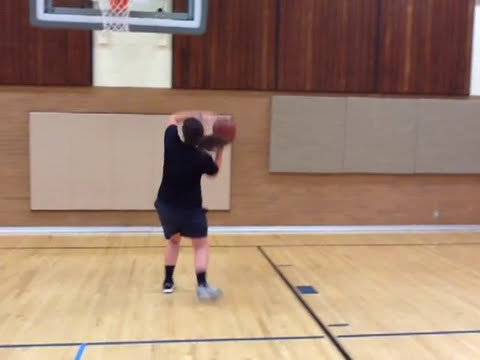In this image, a young boy with long, dark hair tied in a ponytail is captured in the midst of shooting a basketball with his right hand toward a hoop mounted on a brown wooden-paneled wall. He stands slightly off-center to the left on a polished, light wood gymnasium floor adorned with blue and black markings. The boy is dressed in a black t-shirt, blue shorts, gray sneakers, and black socks. The background features a detailed brown wall with gray and tan padding at the bottom, culminating in horizontal wood paneling near the ceiling where the basketball hoop is mounted. The upper left section of the image shows part of a white-bordered backboard with the attached net. Although the still appears blurry and pixelated, the hustle and action of the moment—captured on a low-quality video—remain clear.